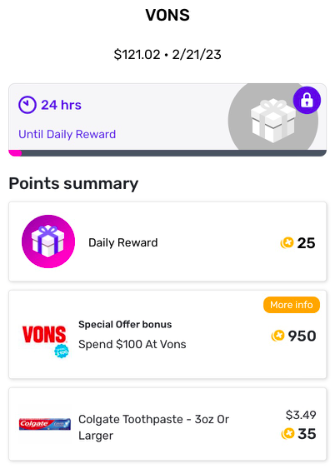Here is a cleaned-up and detailed caption for the image described:

---

This is a smartphone screenshot displaying approximately half of a web page from VONS. At the top of the page, the VONS logo is prominently shown. Directly below the logo, there is a numerical figure of $121.02, followed by a sequence that appears to be a date: 21/23. 

Beneath this, there is a box featuring a clock icon with a message indicating "24 hours until daily reward." To the right of this message, there is an image of a wrapped gift box secured with a lock. 

Further down the page, a section titled "Points Summary" is visible, listing three vertical entries:

1. The first entry has an icon of a white gift box with a purple ribbon and the label "Daily Reward," earning 25 points.
2. The second entry repeats the VONS logo with a sky-blue sticker below it, though the text on the sticker is unreadable. The entry reads "Special Offer Bonus" in black text, with the guideline "Spend $100 at VONS" next to a "More Info" tab on the right, and a points value of 950 listed.
3. The third entry pertains to "Colgate Toothpaste," specifying it must be 3 ounces or larger and priced at $3.49. This entry is associated with 35 points.